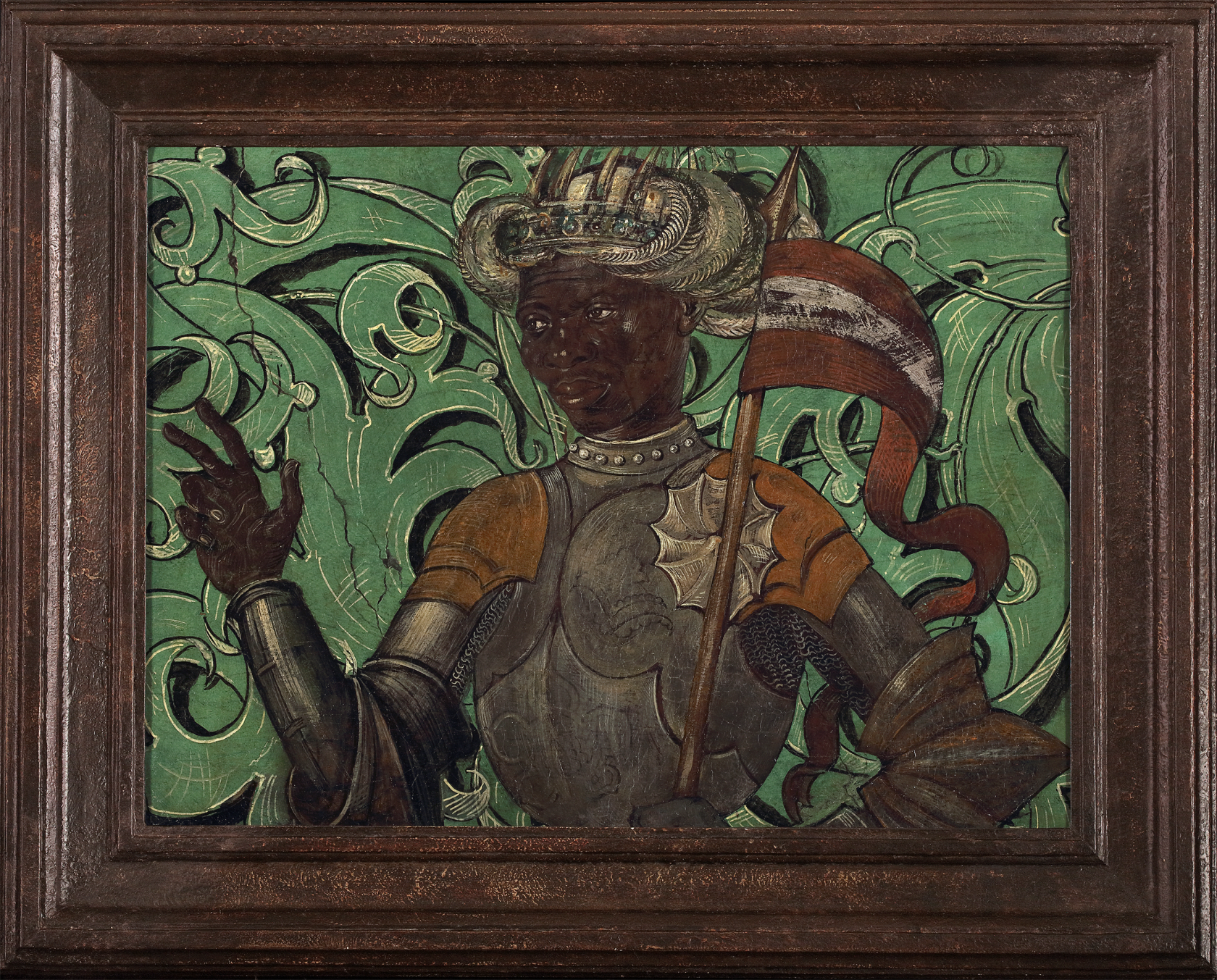This photograph captures a rectangular painting housed within a thick, dark brown wooden frame, which measures approximately one inch wide and features a tiered design with pockmarks indicative of age. The frame surrounds an intriguing image with a greenish background that contains swirls evoking leaves or banners.

The central figure, an African American man depicted from the waist up, appears regal and noble. He dons intricate metal armor with orange shoulder plates and silver body plating. On his head, he wears an ornate helmet adorned with curled feathers and embellished with gold, green jewels, and what looks like large teeth at the front. His left arm is bent at the elbow, holding a spear with a red and white flag or banner. His right hand is raised, with his index, middle finger, and thumb extended in a gesture similar to a peace sign, while his ring and pinky fingers are folded down. The overall composition radiates a sense of historical grandeur and complex character.